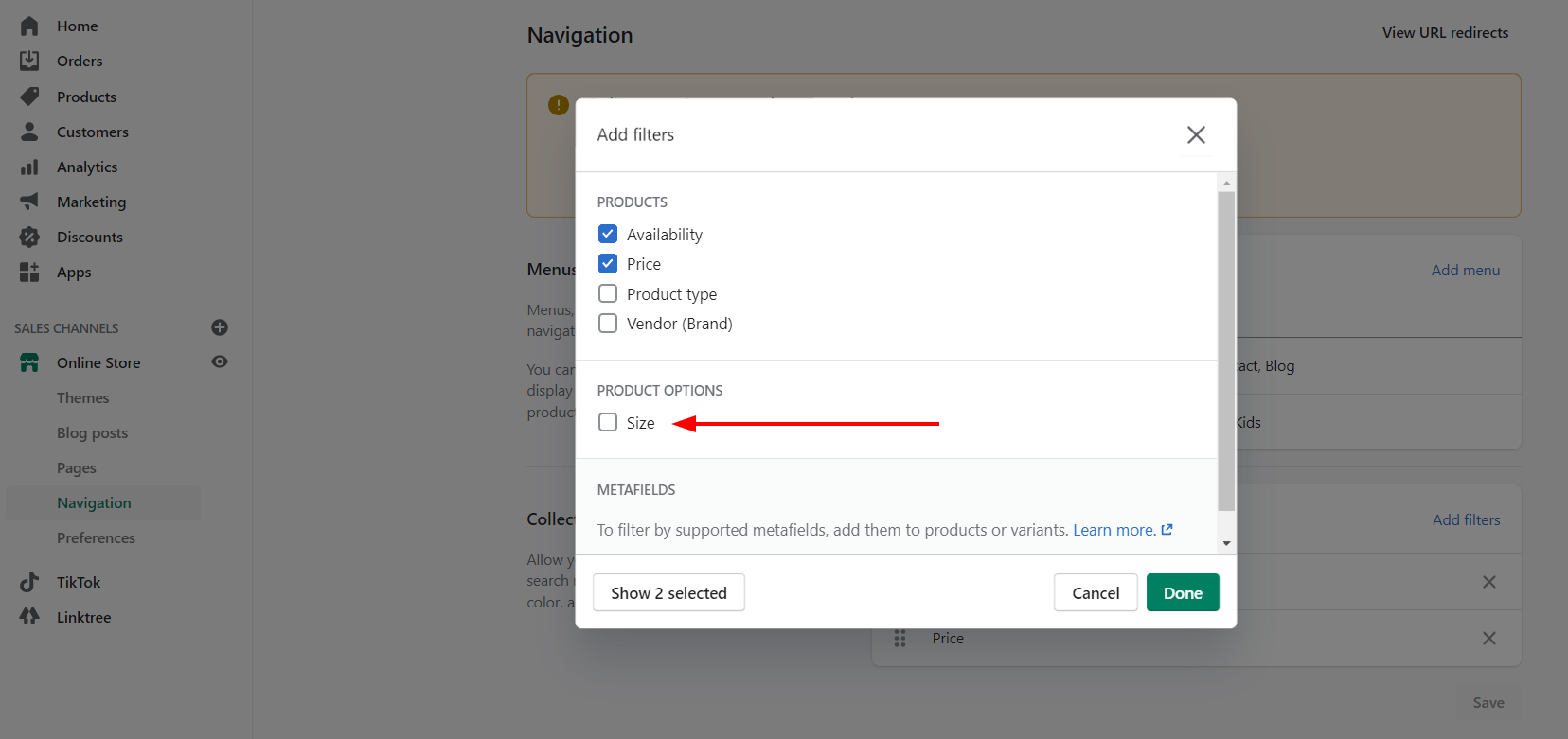This image shows a computer monitor screen in landscape orientation, displaying a web interface of an online store, which is partially grayed out. At the center of the image is a prominent white square dialog box with various options and information.

In the foreground, at the top-left corner of the white dialog box, is the text "Add Filters" while the top right features an 'X' button for closing the box. Below this is a subheading “Products,” followed by four square choice boxes labeled "Availability," "Price," "Product Type," and "Vendor" (parentheses "Brand"). Both "Availability" and "Price" are highlighted in blue with white check marks indicating they are selected.

Further down, the dialog introduces another section titled "Product Options," accompanied by a square choice box to select “Size,” which is visually emphasized by a red horizontal arrow, pointing from right to left, towards the word "Size."

The screen transitions to a gray section below, which contains the text: "Metafields to filter by supported metafields, add them to products or variants," followed by a clickable link labeled "Learn more." Towards the bottom of this dialog box are three buttons: "Show 2 selected" (left), "Cancel" (middle), both in white with black text, and "Done" (right), a green button with white text, situated at the bottom right.

In the background, the larger grayed-out screen features a column of navigational options along its left side, each paired with an associated icon. From top to bottom, these options are: Home, Orders, Products, Customers, Analytics, Marketing, Discounts, Apps, Sales Channel, Online Store, Themes, Blog Post, Pages, and Navigation, which is highlighted in green. Below, other options listed in dark text include Performance, TikTok, and Linktree.

In the central part of the grayed-out panel, the heading "Navigation" is displayed in bold at the top. To the top right of this section is a link labeled "View URL Redirects." Below these, the options "Menus" and "Filters" are partially visible but are mostly obstructed by the white dialog box.